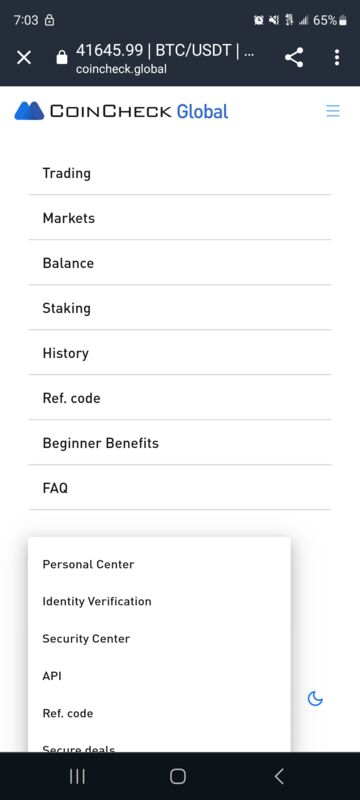In the image, the background is white. At the top, the time is displayed as 7:03, with the battery and alarm icons nearby. The interface prominently features the "Coin Check Global" logo, which includes two blue triangles and the word "Global" in blue. A blue hamburger menu icon is visible as well. Below this, a list of options includes "Trending Markets," "Balance," "Staking," "History," "Ref. Code," "Beginner Benefits," and "FAQ." 

A white box houses additional options such as "Personal Center," "Identity Verification," "Security Center," "API," "Ref. Code," and "Secure Deals." To the right of this box, there's an outline of a moon in blue.

At the bottom of the screen, a black rectangle features icons: three horizontal lines, three vertical lines, a square, and a less-than symbol.